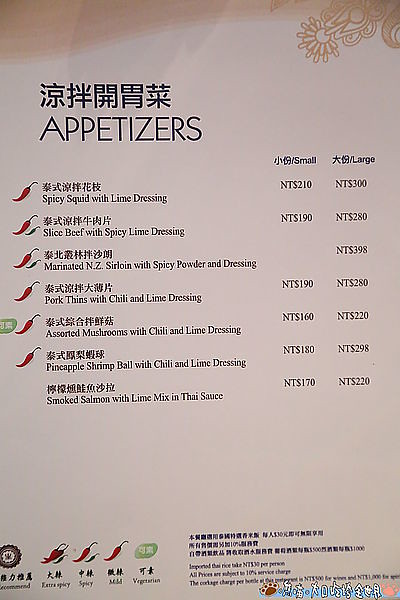The image is a color photograph of a menu page from an Asian restaurant, displayed in portrait orientation. The background of the page features a pale beige-pink hue with a swirl pattern and flower outlines in the top right corner. The menu is tilted slightly, with the right side elevated. At the top left, in bold black text, the heading "APPETIZERS" is prominently displayed in both English and Asian characters. 

Beneath the heading, the menu lists several dishes vertically down the left-hand side, each with red chili pepper icons indicating spiciness. The listed items include:
1. Spicy Squid with Lime Dressing – Small: $210, Large: $300
2. Sliced Beef with Spicy Lime Dressing – Small: $190, Large: $280
3. Marinated New Zealand Sirloin with Spicy Powder and Dressing – Large only: $398
4. Pork Fins with Chili and Lime Dressing – Small: $190, Large: $280
5. Assorted Mushrooms with Chili and Lime Dressing – Small: $160, Large: $220
6. Pineapple Shrimp Ball with Chili and Lime Dressing – Small: $180, Large: $298
7. Smoked Salmon with Lime Mix in Thai Sauce – Small: $170, Large: $220 (without a chili pepper icon)

To the right of the dish names are the corresponding prices for small and large portions, arranged in two separate columns. 

At the bottom of the menu, a spiciness legend explains the chili pepper symbols: one pepper for mild, a red and green pepper for spicy, and two red peppers and one green for extra spicy. The bottom right corner features additional text in Asian characters, with English translations beneath, though they are too small to be legible in the photograph. The menu's overall design and detailed illustrations emphasize a photographic realism style.